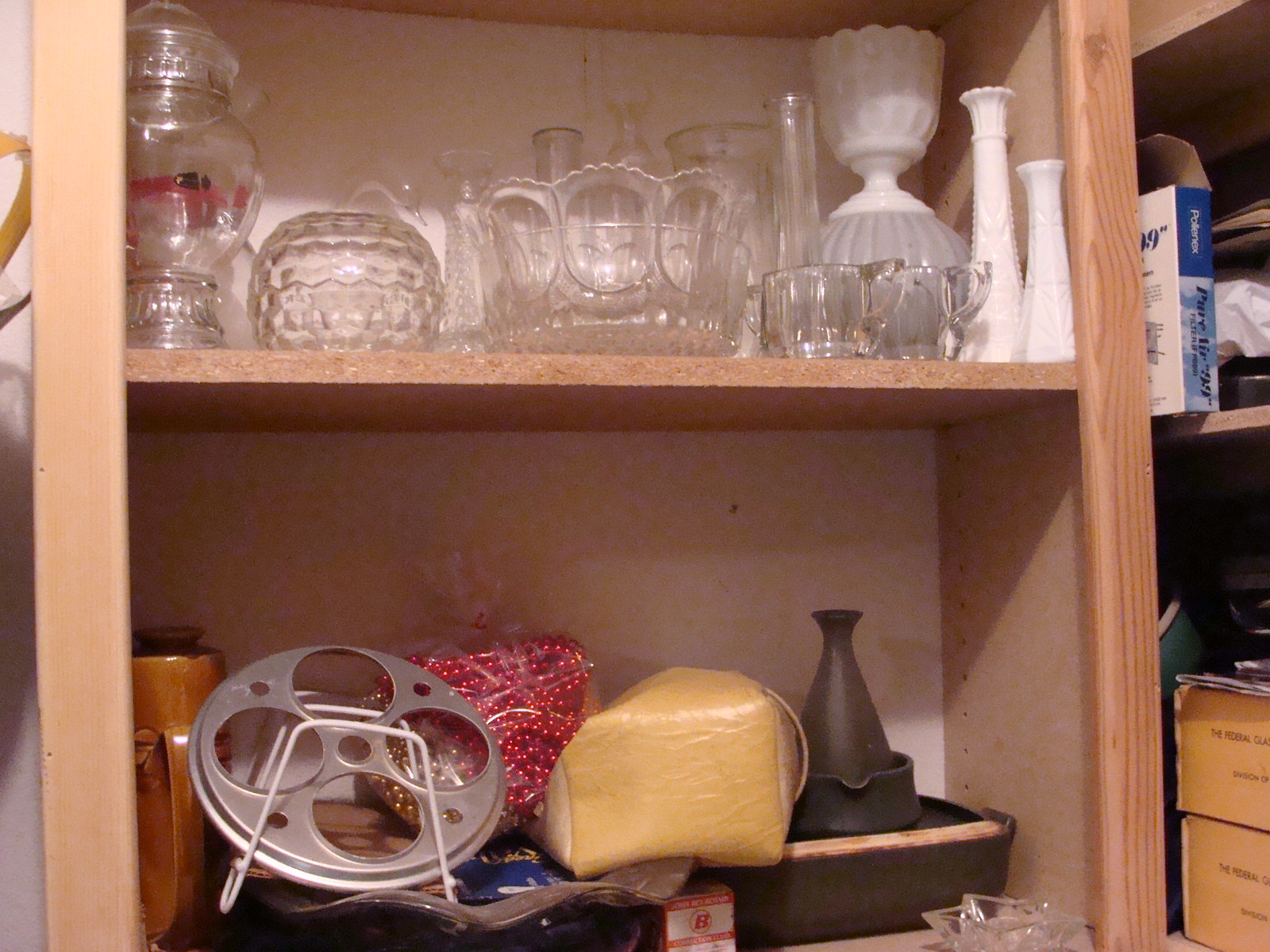In the image, we see an intricately detailed brown wooden hutch. The top shelf features a rich wooden texture on its bottom and side panels. On this shelf, a collection of elegant crystal pieces is displayed prominently. Among the crystal collection is a taller, slender crystal jar, a smaller round crystal jar, and an elevated crystal bowl. Also on this shelf are two short glass mugs and two white tapered candlesticks, adding to the eclectic mix of items.

The second shelf from the left offers a glimpse of a light brown tiki cup's side, showcasing the area designed for holding the cup. Adjacent to this is a vintage movie reel, characterized by its silver color, with four large and four smaller circles within it. A plastic bag filled with vibrant red beads is also visible, along with the yellow end of a purse. Additionally, a piece of brown home decor—possibly a vase—can be seen. Below this, to the right, sits a small, delicate crystal ashtray.

On the far right of the hutch, there are the edges of several brown books stacked neatly. Positioned above these books is another book with a distinctive blue binder, rounding out the diverse array of objects arranged on the shelves.